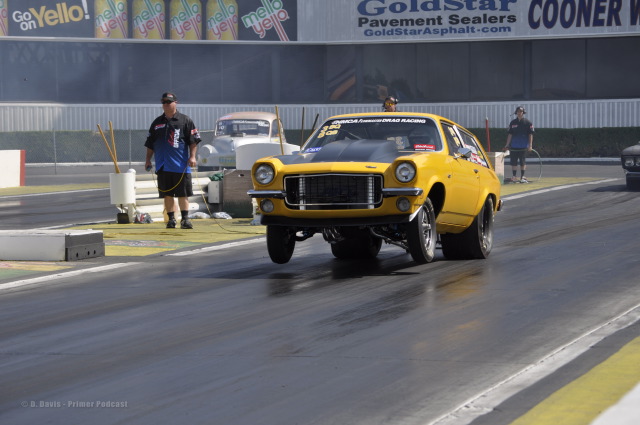The image captures a dramatic moment at a drag race on what appears to be a quarter-mile track. The black track surface, which looks slightly shiny and possibly wet, stretches diagonally from the right side of the picture to the lower left. Dominating the scene is a heavily modified yellow car, likely an older model hatchback from the 70s, characterized by its blocky, angular design and distinctive black hood with a significant curve and lift hinting at a powerful engine. The car's large Mickey Thompson rear tires and thin front wheels underscore its rear-wheel-drive configuration optimized for drag racing. The car is in the midst of launching from the starting line, its front wheels lifted off the ground, indicating a powerful acceleration. Surrounding the track are several individuals, including a man in a blue shirt and black shorts, possibly officials or pit crew members, overseeing the race. Visible sponsor logos, such as Mello Yello and Gold Star Pavement Sealers, add to the authentic drag racing atmosphere.